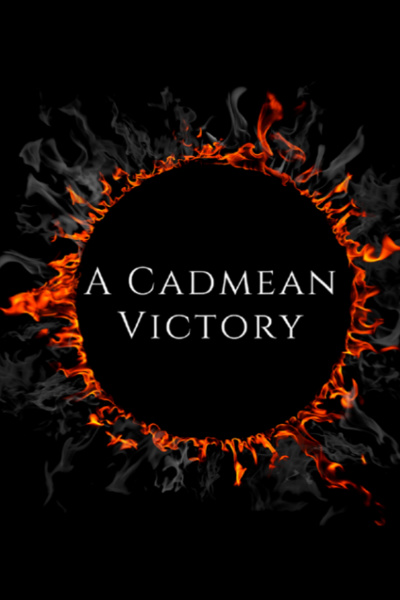The image features a dramatic and intense visual composition suggestive of a celebratory or victorious event. It is a vertically aligned rectangular digital illustration set against a completely black background. Dominating the center of the image is a large, vibrant ring of fire with red-orange flames of varying sizes emerging outward. The longest and widest flame appears around the nine o'clock position, while the flames between the ten o'clock to noon region are the smallest. Enveloping this fiery ring is a layer of gray smoke that expands outward, creating a smoke ring effect.

At the very core of this spectacle, in bold white capital letters, the words "A CADMIEN" are prominently displayed, stretching horizontally across the center. Directly beneath this, also in bold white capital letters and in a slightly spaced-out format, is the word "VICTORY". This structured typography commands attention and attributes a sense of significance and grandeur to the text. The words and the fiery ring are centrally placed, effectively stretching from the top to the bottom and touching the sides of the image. The overall design is striking and symbolic, creating a powerful visual statement.